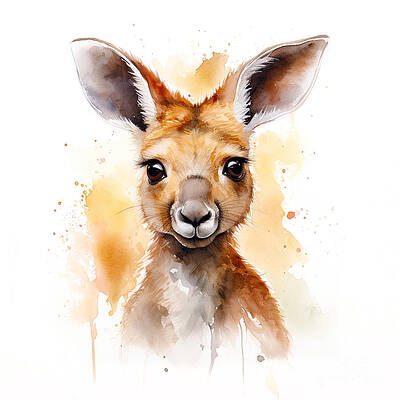This captivating image showcases an AI-generated watercolor painting of a baby kangaroo, depicted in a slightly cartoonish style. The scene focuses on a headshot of the joey, capturing it from its neck up with its glossy, expressive dark brown eyes and short, upright ears presenting an innocent and endearing look. The fur of the kangaroo is rendered in a blend of beige to brown-reddish hues, and subtle details like eyelashes enhance its charming appearance. The background is primarily white, adorned with splashes and drips of light brown, orange, and yellow watercolor, giving the impression of a dynamic and artistic backdrop. The overall composition emphasizes the kangaroo's endearing gaze and soft features, blending seamlessly with the lively watercolor effects.